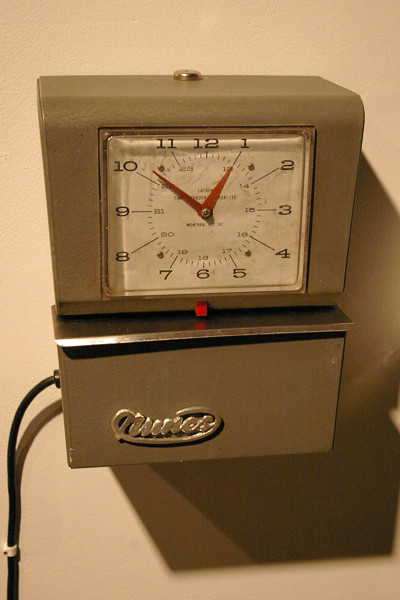On the wall, there is an industrial-style clock with a distinctive setup. The clock itself is encased within a square glass window. It has a white face adorned with black numerals and lettering, while its hands are constructed from red metal, showing the time as 10:51. Attached below the clock is a shiny, light brown or light gray metal box, notable for its rectangular shape and stainless-steel finish. The box features a lid and has a cursive logo on its front, though the brand name is indiscernible. Extending from the side of the metal box is a black power cord, which is securely fastened to the wall several inches below using a white plastic bracket.